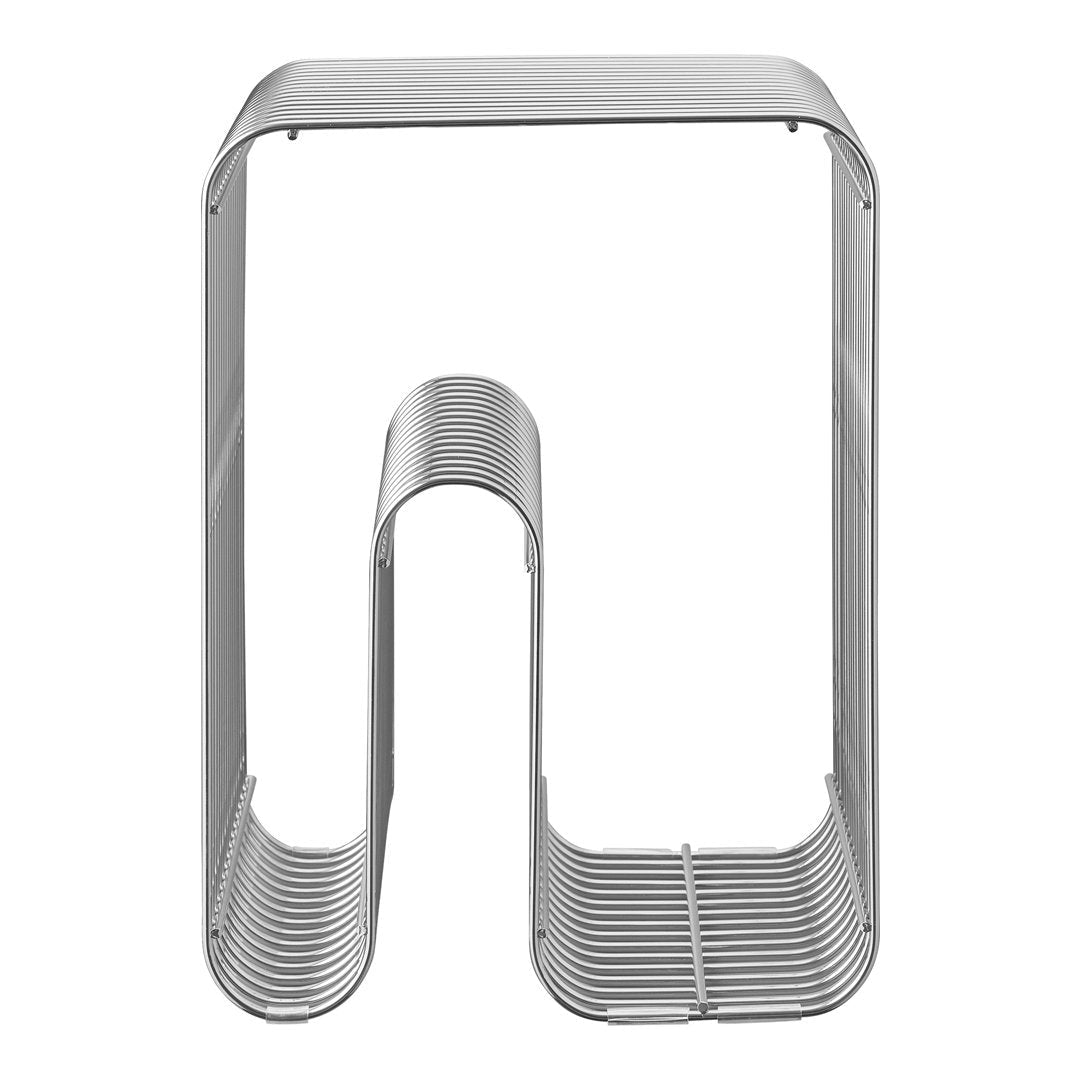The image depicts a sleek, modern letter or folder holder made of thin, tubular metal bars, likely stainless steel, arranged horizontally with a vertical orientation. Resembling a minimalist sculpture, the device features over a dozen parallel bars weaving through a continuous frame, devoid of any breaks or ends. Centrally positioned on a white background, the holder’s design includes a unique, curved section at the base that forms arch-shaped compartments intended to organize and hold envelopes or files. The arrangement of the metal bars, with their rounded edges and precise alignment, creates a visually striking, open structure, accentuated by the photograph's clean, product-centric style.